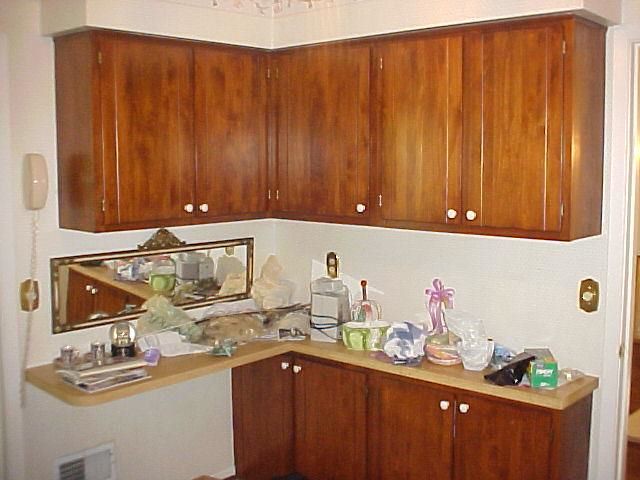The photograph captures an indoor color image of a cluttered kitchen corner from what appears to be an early 1980s or late 1970s decor. The upper portion features L-shaped wooden cabinets with white knobs, stained in a dark brown hue, hanging from the ceiling. The countertop below is tan-colored laminate, similarly flanked by L-shaped cabinets on the lower half that match the upper ones. The countertop is strewn with various items, including a snow globe, ceramic bowls, soap, tassels, and even a stapler. A small mirror is affixed to the wall above the countertop. To the left side of the image, there's a wall phone with a white cord and a dimmer switch with a gold plate beneath it. On the right, another dimmer switch with a gold plate is visible next to the edge of a door frame. This kitchen scene, loaded with an eclectic mix of items, suggests a space that is both nostalgic and lived-in.